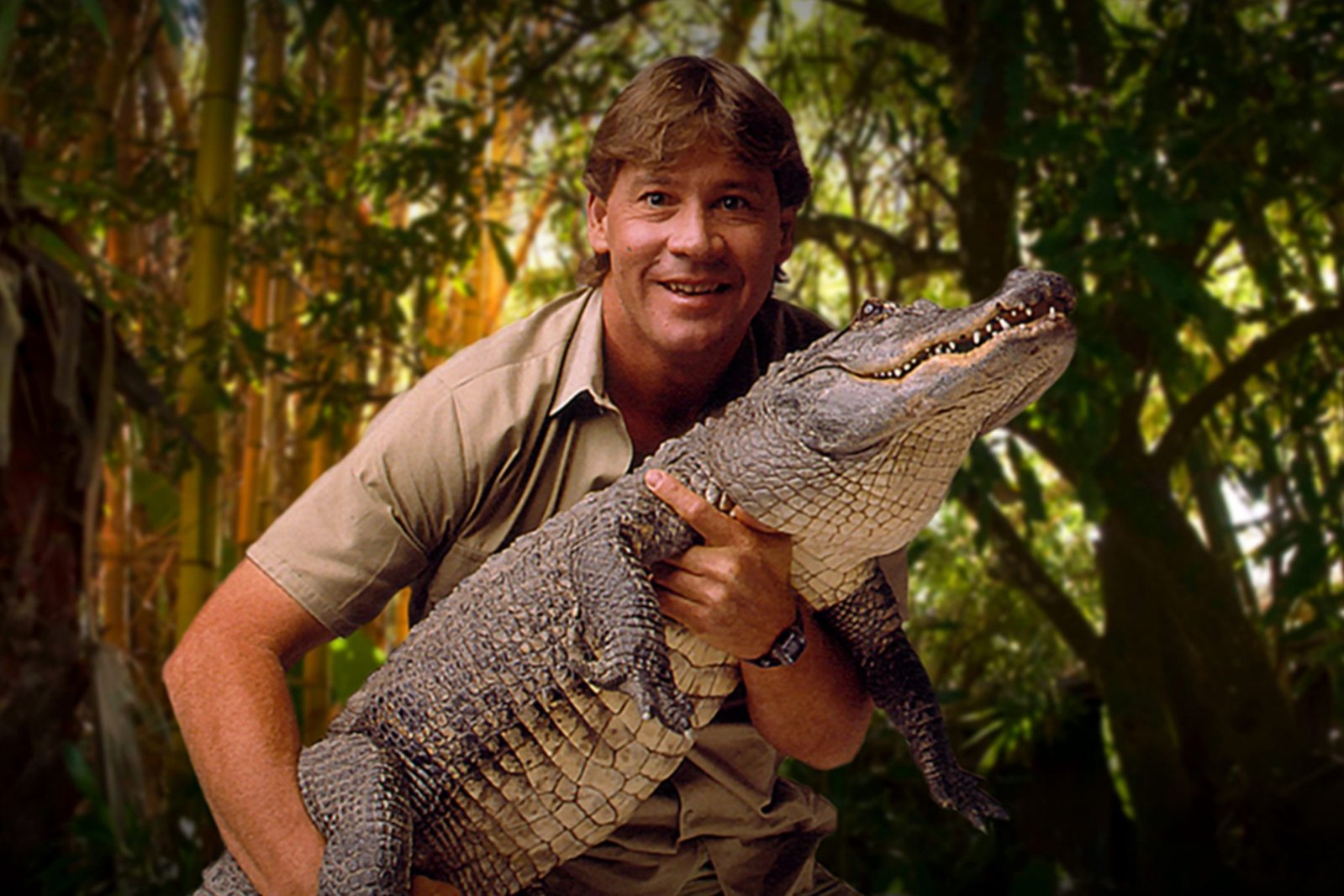In the image, a man resembling the famed animal expert Steve Irwin is prominently featured. Steve, known for his work with animals and his popular wildlife shows, stands confidently with a broad grin directed at the camera. His iconic light tan, collared shirt and shorts are unmistakable. Steve exhibits his characteristic enthusiasm, holding a sizable alligator (or possibly a crocodile) with ease. 

In the photo, Steve's tanned complexion is highlighted, and his characteristic brown, slightly mullet-styled hair adds to his familiar appearance. He is wearing a watch on the hand that's placed under the reptile’s neck, while his other hand grips its tail. The alligator, appearing quite unfazed and calm, is cradled comfortably in his arms. 

The background evokes a dense, dark jungle or rainforest setting, although the contrast between the brightly lit Steve and the shadowy surroundings suggests a potential photoshop enhancement. The left side of the image showcases tall bamboo shoots, while the right side features thick jungle trees. An obscure, darker sky fills the center, further emphasizing the lush and exotic environment around him.